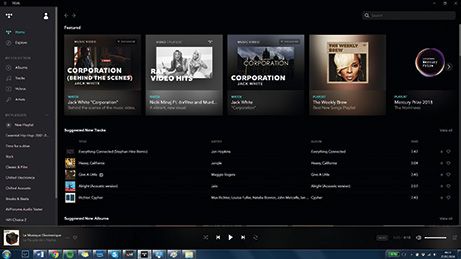This is a screenshot of an unidentified music website. The interface features several distinct sections, although much of the text is too small and blurry to decipher. At the top of the webpage, there is a prominent piece of cover art titled "Corporation Behind the Scenes, Jack White Corporation," featuring an individual gazing to the right. Below this, there is a section called "Rap Video Hits," displaying a striking black-and-white photograph of two dark-skinned women. Further down, another section labeled "The Corporation" is shown, followed by a segment titled "The Weekly," accompanied by an indistinct word and an image of an African-American woman who appears to resemble Mary J. Blige, notable for her short blonde hair combed over her left eye. A vertical dropdown menu is positioned on the left side of the page, and numerous icons are aligned at the bottom. No animals, buildings, or airplanes are visible in the screenshot.